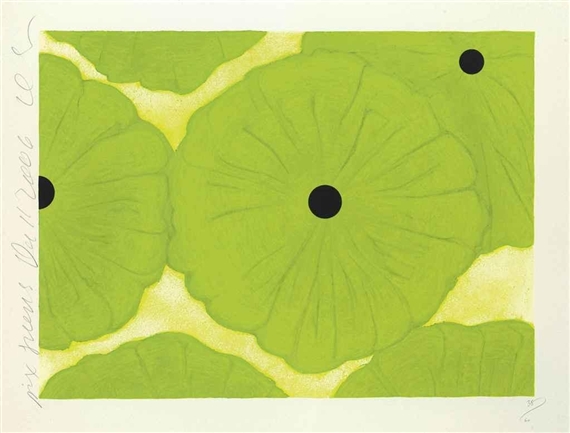The image appears to be an illustration, likely a painting or watercolor, featuring six green, circular flowers with a distinct black center and radiating veins. The flowers are arranged in such a way that only one is fully visible in the middle, while parts of the other five extend beyond the edges of the frame. The artwork is bordered by a light gray border, and there is handwritten text running vertically along the left-hand side in blue, although it's mostly illegible except possibly for the year "2006". The background of the image is a blend of light yellow and white, adding to the illustration's ethereal quality. The piece also includes a signature with what seems to be initials, and it appears to be numbered on the lower right, indicating it might be part of a series or a limited edition.